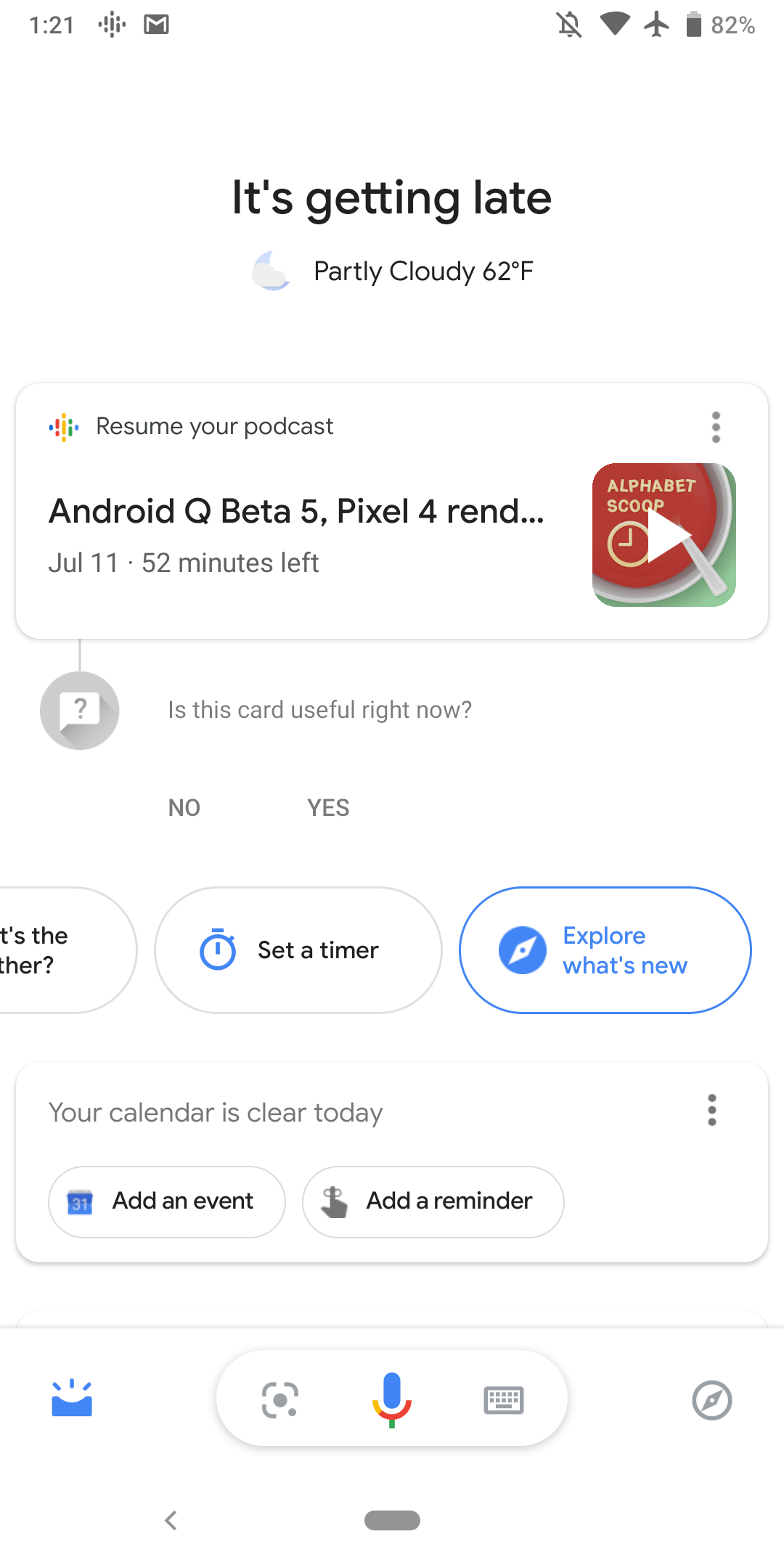The image showcases what appears to be the home screen of an Android phone. At the very top, typical home screen icons are visible, including the current time displayed as 1:21, alongside icons for notifications such as no alarm, Wi-Fi, airplane mode, and a battery indicator showing 82%. The background is predominantly white.

Below these icons, a text message reads "It's getting late," accompanied by a weather icon featuring a moon partially covered by a cloud, indicating a partly cloudy night with a temperature of 62 degrees Fahrenheit.

Further down, there is a section encouraging the user to "Resume your podcast," specifically highlighting "Android Q beta 5, Pixel 4..." with the text truncated by an ellipsis. An image next to this text displays the "Alphabet Scoop" podcast, depicted with a soup-themed background and a clock icon. A play button overlays this image, suggesting users can continue their podcast playback from here. Additional details note "July 11th, 52 minutes left."

Beneath the podcast section, a query asks, "Is this card useful right now?" with options to respond "Yes" or "No." 

The next section offers three selectable options: "Explore what's new" (currently selected), "Set a timer," and "What's the weather." 

Finally, the screen states "Your calendar is clear today," providing options to "Add an event" or "Add a reminder." At the bottom of the screen, more icons are visible, including a microphone, a keyboard, an unknown pointer icon, and a browser icon.